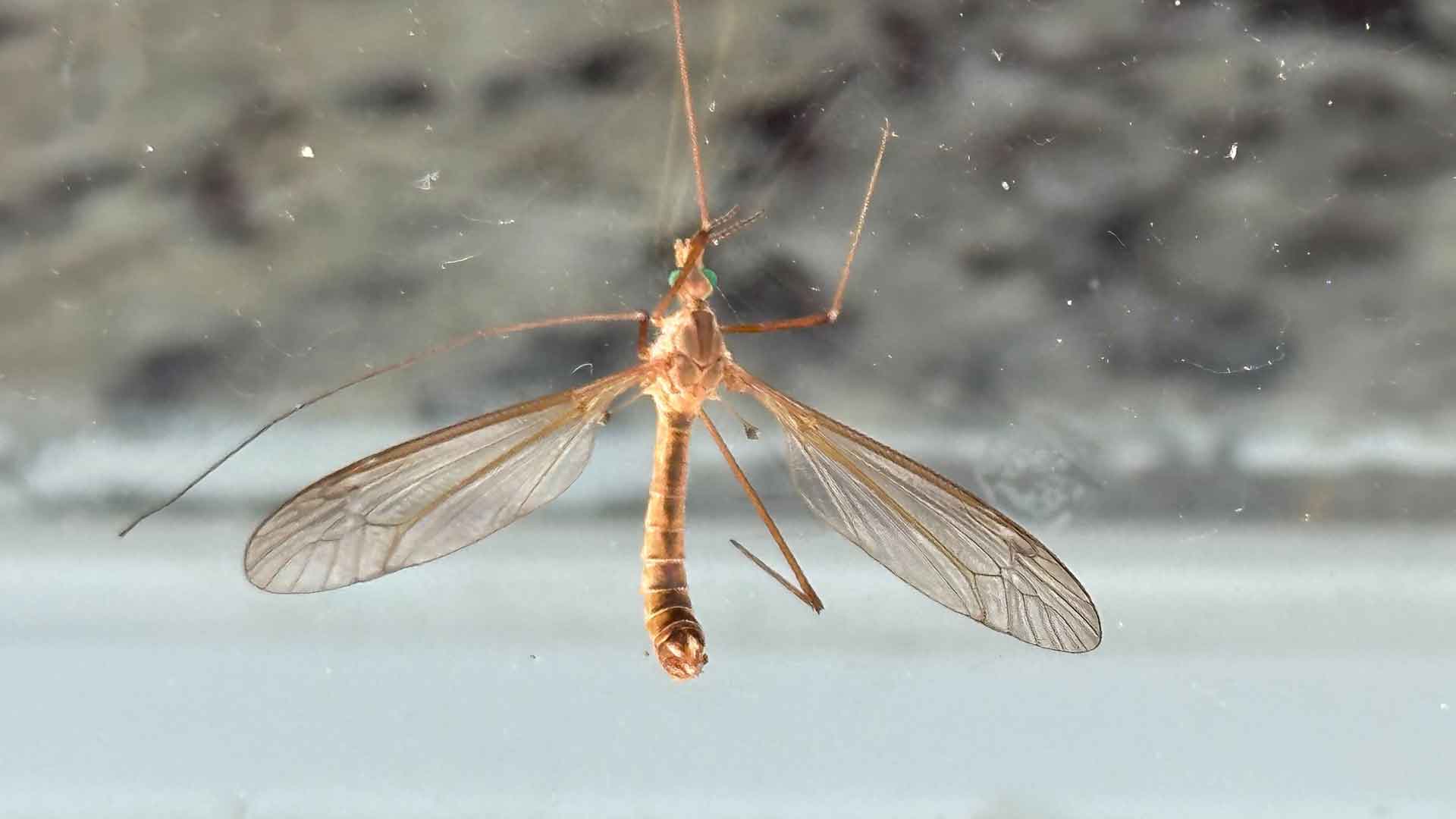A highly detailed close-up of a dragonfly, possibly caught in a spider's web. The insect's wings are fully spread and translucent, revealing intricate vein patterns under the bright sun. The dragonfly, brown with a hint of blue in its eyes, stands out sharply against a significantly blurred background that might include a sky, beach sand, hills, or even water. The background elements are indistinct, possibly seen through a dirty window, further drawing focus to the dragonfly. Despite the slightly unclean glass that adds specks and spots to the image, the dragonfly's legs, tail, and delicate wing structure are captured in remarkable detail, highlighting the fragility and complexity of its form.